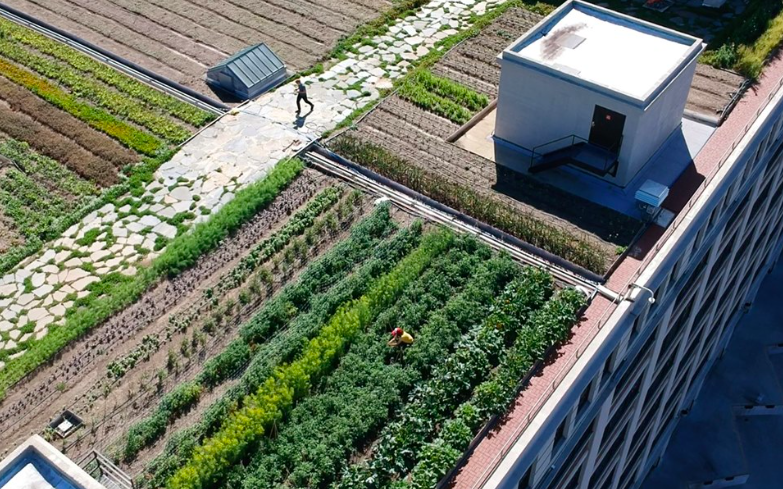This overhead photograph vividly captures a multi-storied building featuring a rooftop agricultural area. The rooftop hosts a variety of green plants, including vegetable and fruit gardens, organized into distinct crop fields. The building itself is primarily white and gray, complemented by black stairs leading to an entrance visible from above. A white stone pathway winds through the lush greenery, which teems with plants sporting a spectrum of leaves from light to dark green. 

Two individuals are discernible in the scene: one is actively working in the garden, donning a red hat, while the other strolls beside the crops along the stone walkway. Additional elements include a brown field and a solar panel, emphasizing the sustainable aspects of the rooftop garden. Some windows on the building's lower right side hint at the structure's expansive size. The photograph also captures the paved area at the base of the building, characterized by a dark gray hue. Bathed in sunlight, this rooftop oasis epitomizes urban agriculture and sustainable design.